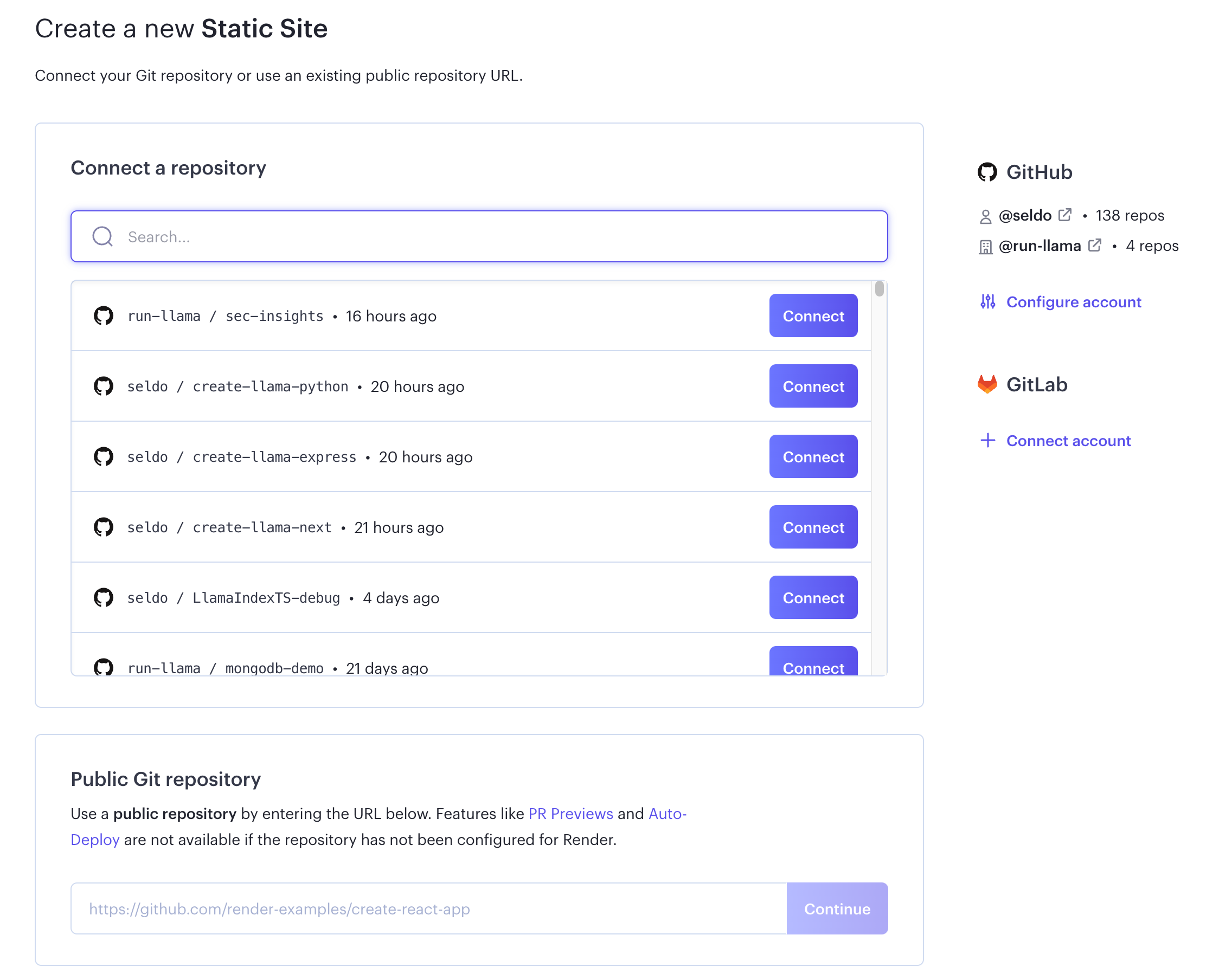The webpage displayed is designed for creating a new static site. At the top, it prompts users to either "Connect your Git repository" or to use an existing public repository URL. Below this, a search bar outlined in blue allows users to find and select their repository. The page lists various repositories, each in a separate box, detailing different programming languages and timestamps indicating updates, such as "16 hours ago," "20 hours ago," "21 hours ago," and "4 days ago." 

Each repository box features a purple "Connect" button on the right side, enabling users to link the repository to the static site creation tool. Under this section, there is an additional prompt to use a public Git repository by entering its URL directly. The page notes that features like "PR reviews" and "Auto-deploy"—highlighted in blue—are unavailable if the repository hasn't been configured for render.

At the bottom of the image, there’s a section labeled "Website," including an example URL field. The "Continue" button next to this example is currently grayed out, indicating it is inactive until further input is provided.